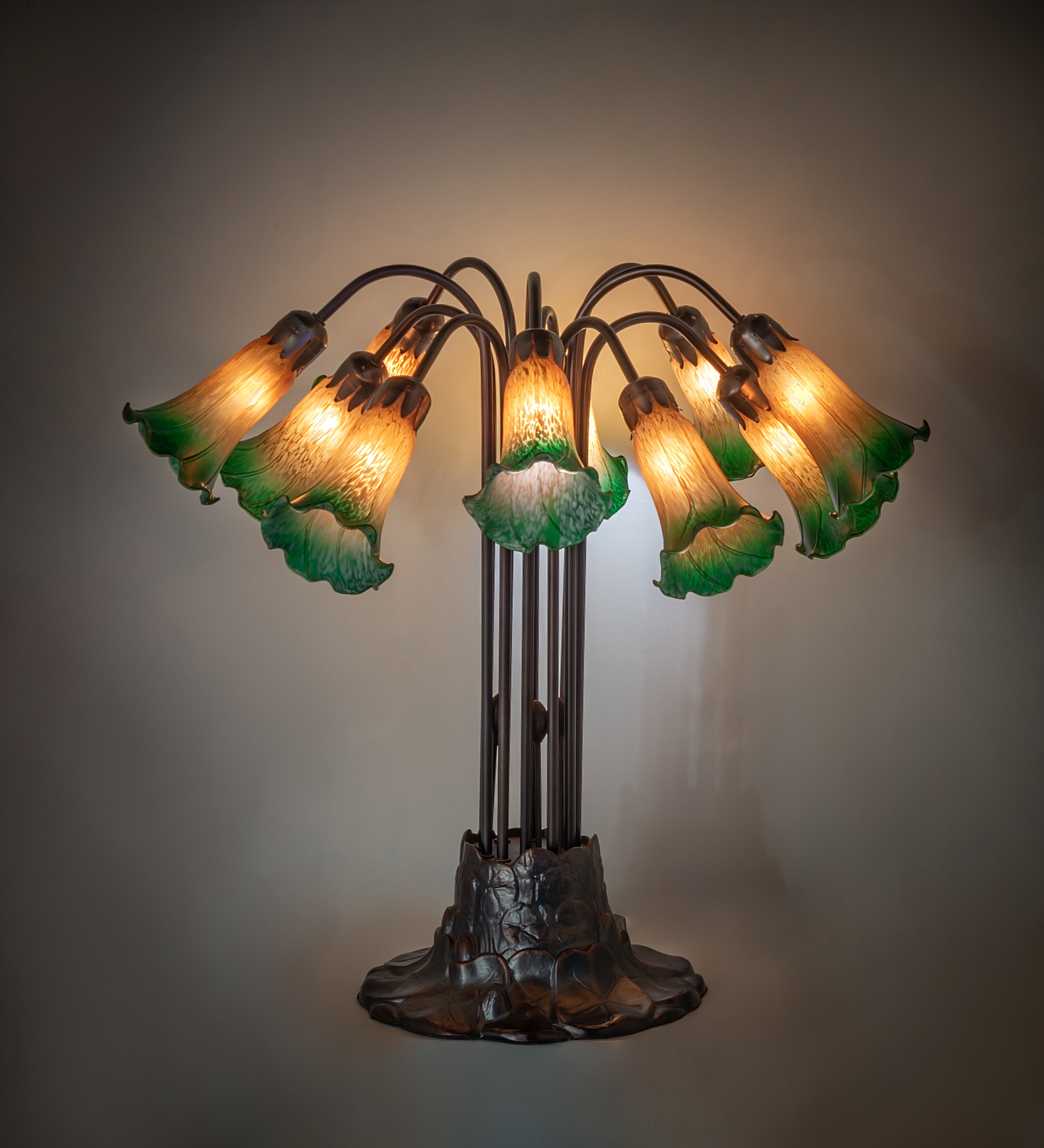The image portrays a unique stand-up table lamp set against a white background in a dimly lit room, giving it a studio-like ambiance. The lamp features a striking design with a base resembling a tree husk or stub, from which several curving poles rise and arch downward. At the ends of these poles, there are ten flower-like lampshades that emit light. These lampshades are predominantly yellow with green tips, creating a vibrant, floral effect. The detailed and multi-featured design of the lamp makes it an intriguing and different centerpiece.